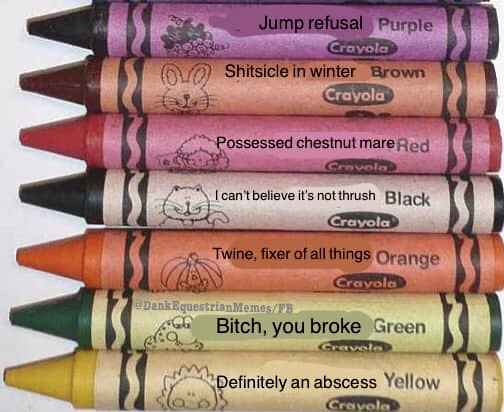The image is a close-up, overhead photograph of seven Crayola crayons meticulously laid out side-by-side, all uniformly sized and pointing to the left. Each crayon bears a humorous, edited label along with a unique drawing on its wrapper. The crayons are stacked in the following order from top to bottom:

1. **Purple Crayon**: With a light purple wrapper featuring a bunch of grapes, it is humorously labeled as "Jump Refusal Purple."
2. **Brown Crayon**: Wrapped in light brown paper and adorned with a rabbit illustration, it is labeled "Shitsickle in Winter Brown."
3. **Red Crayon**: Sporting a lighter red wrapper with an image of a sheep, it’s labeled "Possessed Chestnut Mare Red."
4. **Black Crayon**: Featuring a white wrapper and a cat drawing, it reads "I Can't Believe It's Not Thrush Black."
5. **Orange Crayon**: Enclosed in light orange paper and illustrated with a pumpkin, it is humorously named "Twine, Fixer of All Things Orange."
6. **Green Crayon**: Wrapped in light green paper with a frog drawing, it carries the label "Bitch, You Broke Green."
7. **Yellow Crayon**: In a light yellow wrapper featuring a sun drawing, it is labeled "Definitely an Abscess Yellow."

Each crayon retains the Crayola logo prominently beneath the whimsical names.